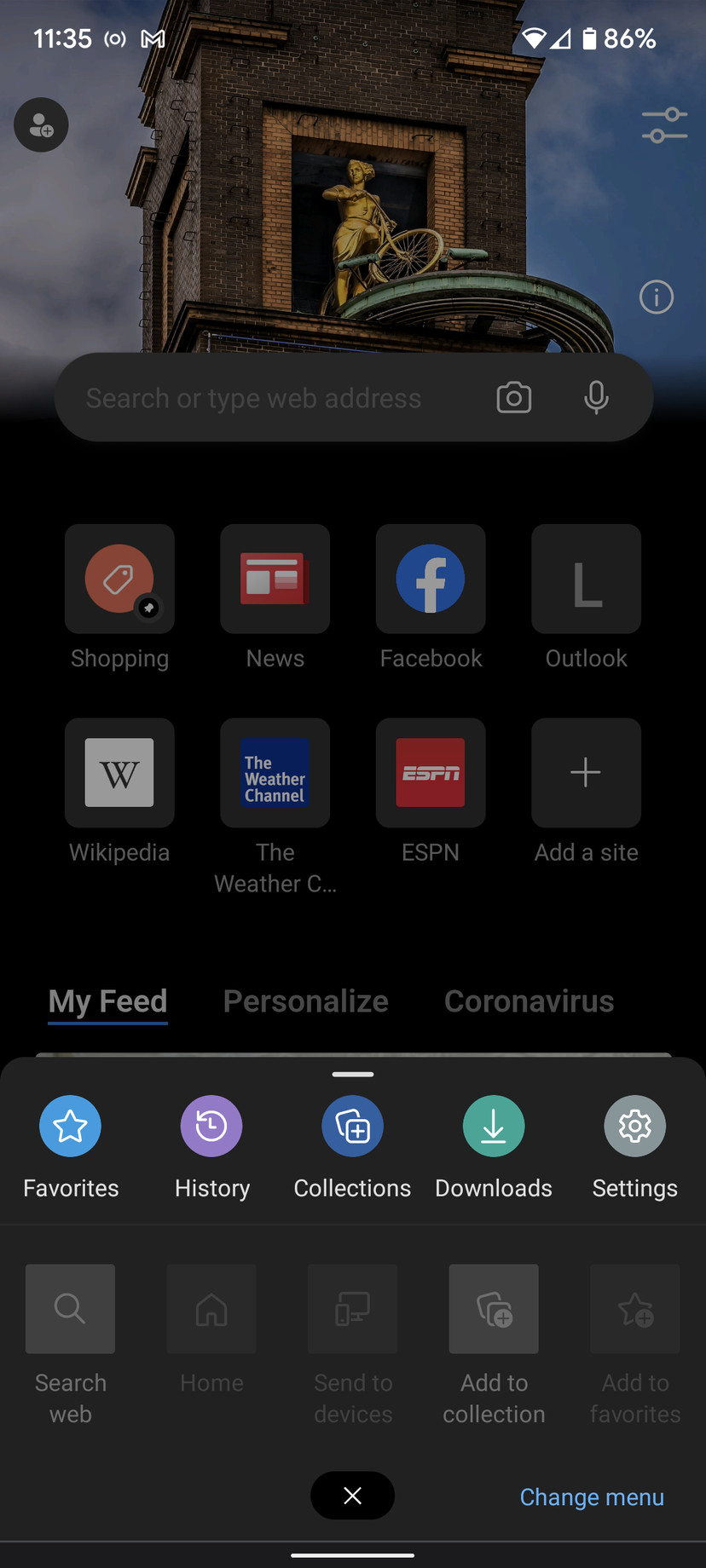The image is a screenshot taken from someone's phone screen with a predominantly black background. In the upper section, a faint outline of a brick building's top is visible, along with a gold statue icon positioned in the middle of a square area. The gold statue appears to depict a figure capable of riding a bike.

Displayed at the top of the screen is the current time, 11:35, and the phone’s battery level at 86%. Below this, a search bar is presented with the text "Search or type web address," accompanied by icons for a camera and a microphone on its right.

Navigating further down, there are several icons arranged in two rows. The top row includes:
- An icon labeled "Shopping" with an associated image.
- An icon for "News."
- The Facebook app icon marked by an "F."
- The Outlook app represented by an "L."

In the second row, the icons include:
- The initial "W" representing Wikipedia.
- A box indicating "The Weather Channel."
- A red box with the text "ESPN" for the ESPN app.
- An option labeled "Add a Site" accompanied by a plus symbol.

Towards the bottom, the screen displays links for "My Feed," "Personalize," and "Coronavirus," followed by more content that extends further down the screen.